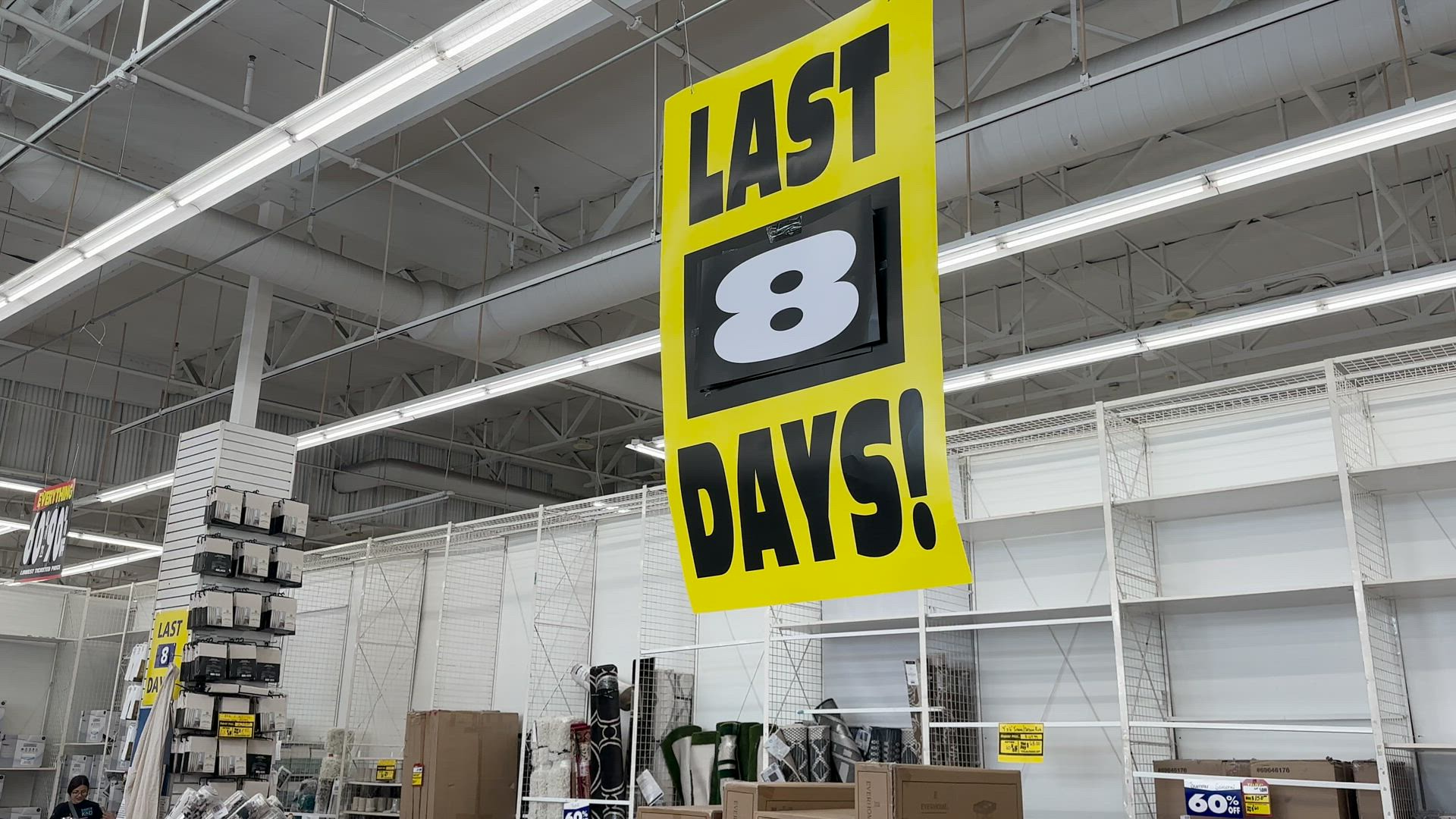The photograph captures the interior of a store, likely a warehouse given the unfinished ceiling with visible conduit and heating ductwork among metal rafters. The ceiling is equipped with long white fluorescent lights running in rows, casting a stark brightness across the scene. The store itself is dominated by white tones, from the walls to the white-painted metal shelves, some of which stand empty. 

Hanging prominently from the ceiling joists is a large, rectangular yellow sign with bold black text that reads "Last Days." The words "Last" and "Days" are separated by a black box containing a large white number "8," which signifies “Last 8 Days.” This number appears removable, presumably to count down the remaining days of a sale. A smaller sign with the same design is affixed to a pillar surrounded by other shelves.

Additional details include signs indicating a "60% off" discount, displayed on blue backgrounds with white lettering. Among the unclear products on display, some rolled-up cylindrical items are discernable and possibly rugs, given their gray and white colors. Against one wall, an opening reveals brown flat cardboard packages leaning against each other. Sporadically placed yellow sale signs adorn the shelving units.

Towards the far edge of the image stands a partly visible individual with white skin, dark hair, glasses, and wearing a black top with a gray strap over the shoulder. The person is a small yet notable element in this detailed depiction of a store in its final sale days.